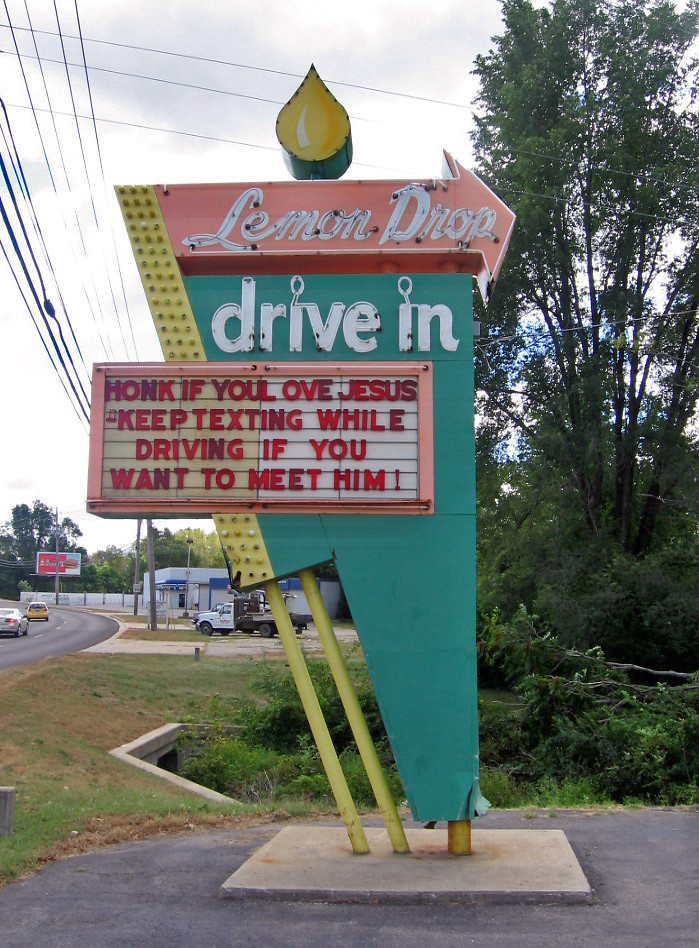This is a color photograph capturing a retro-style sign for the Lemon Drop Drive-In, which boasts a mix of bright, faded, and pastel colors indicative of its age. The sign's prominent features include a vertical yellow section on the left dotted with light bulbs, a bold pink arrow pointing to the right adorned with a lemon-shaped cutout at the top, and a turquoise main body. The words "Lemon Drop" are written within the pink arrow, while "Drive-In" follows beneath in similarly vibrant hues. Beneath this, there is a changeable-letter marquee that reads, "Honk If You Love Jesus. Keep Texting While Driving If You Want To Meet Him," serving as a humorous social commentary on texting and driving.

The sign is mounted on cement, standing on patchy green grass. In the background, there is a mix of trees, power lines, and cars driving on a curving road to the left. A gas station with a white truck parked near it, as well as a billboard—possibly for Arby's—adds context to the setting. Overall, the vintage and somewhat weathered sign juxtaposed with the surrounding elements creates a nostalgic and whimsical snapshot.